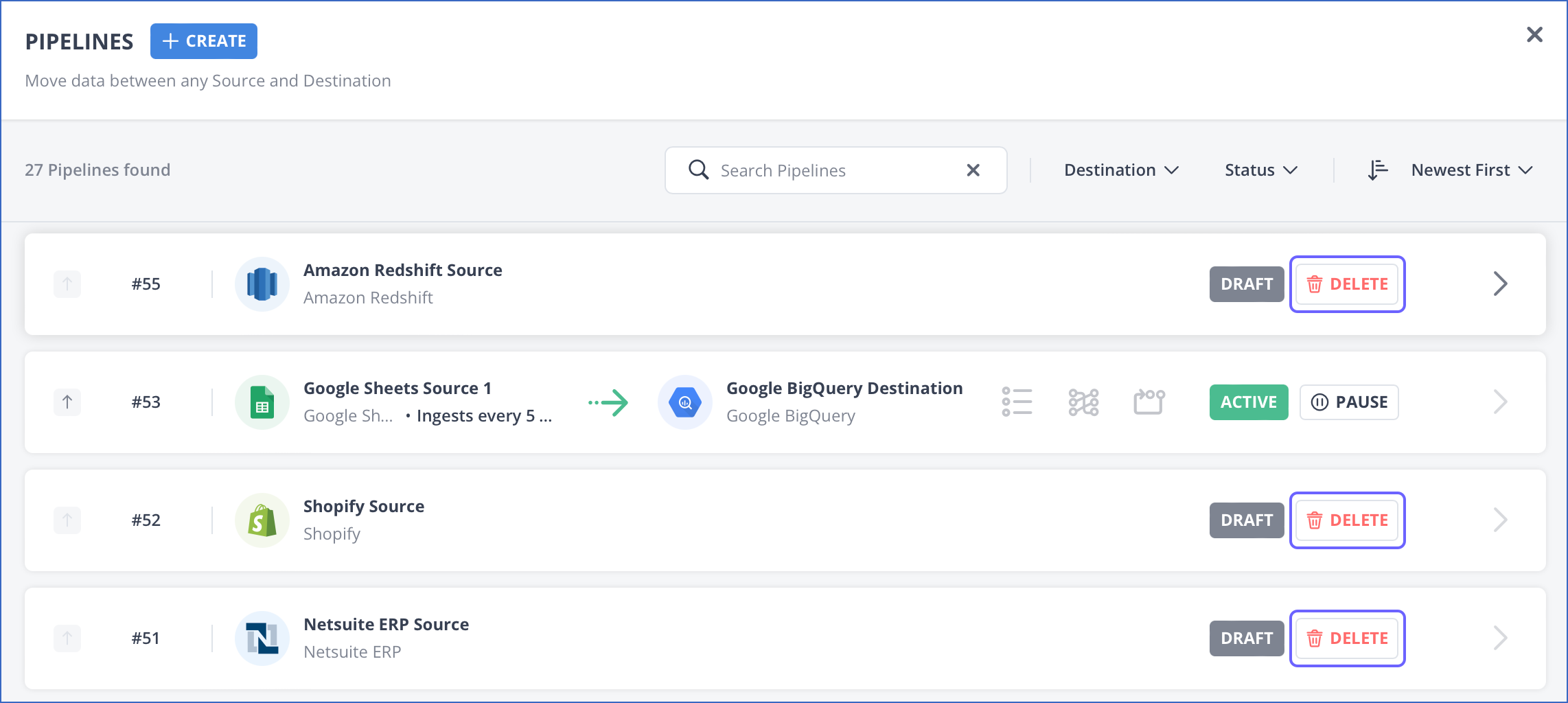The interface is enclosed within a prominent blue-bordered square, with a white interior. In the upper left corner, the word "Pipelines" is displayed. Adjacent to it, a blue box contains a plus symbol, and beside that, the word "Create." Below this header, in light gray text, is the phrase "Move data between any source and destination." Underneath, it states "27 pipelines found." To the right, there is a search bar with the placeholder text "Search Pipelines" in light-colored text.

Horizontally across the interface, there are sorting options labeled "Destination," "Status," and "Newest First." The foremost pipeline entry is labeled "55, Amazon Redshift source," with options to either "Draft" or "Delete," the latter being in red text. Next is "Google Sheets source one," marked as "Active" within a green box. Below this is "Shopify source," accompanied by options in gray text for "Draft" or red text for "Delete." Finally, "Nestitute ERP source" is listed, with options on the right to "Draft" (gray text) or "Delete" (red text) in a blue-outlined box.